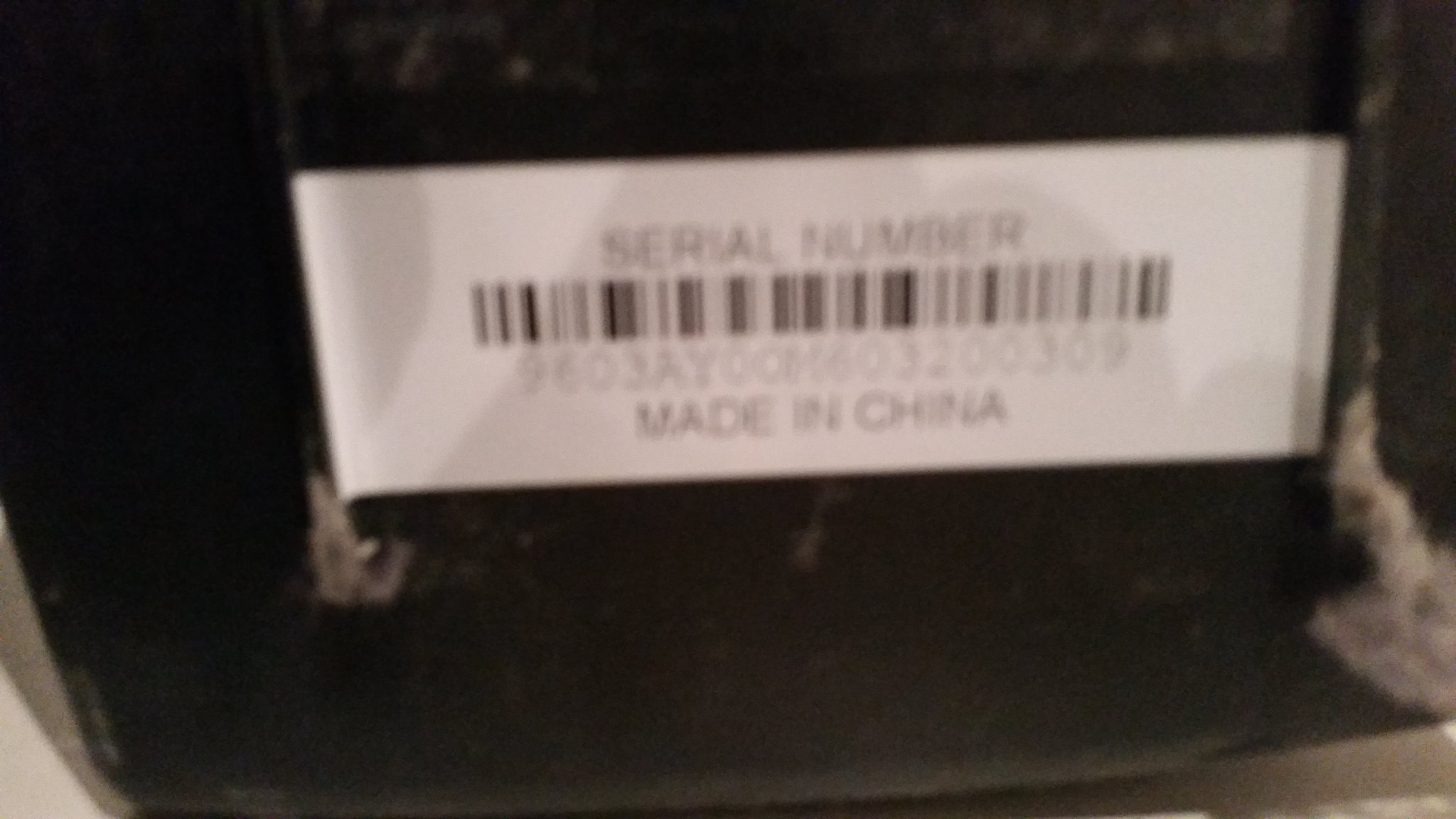This is a close-up, landscape-oriented photograph of a product label, providing a highly detailed yet blurred view. The product itself is black and indiscernible, while the label, a long, wide white rectangle, stands out prominently. Centrally placed at the top of the label is the text "Serial Number." Directly beneath it, a long, skinny barcode stretches horizontally across the label. Below the barcode, a string of approximately 20 digits is partially legible, though the blurriness obscures most of the numbers. At the bottom of the label, the text "Made in China" is clearly visible.